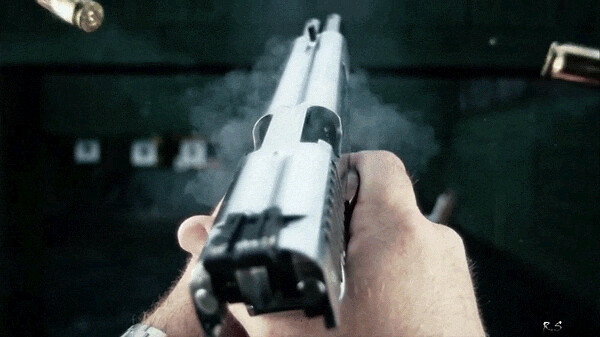In this detailed photograph taken at a shooting range, we see a close-up of a white male's hands firmly gripping a silver and black gun. The right hand is pulling the trigger, visible in the act of firing, as a burst of white smoke emanates from the barrel. The motion captures a remarkable moment—the ejection of spent cartridges, with two bullets visibly flying away from the top sides of the gun. The background is predominantly black, suggesting a dark indoor setting with minimal distraction. Faintly in the distance, on the left-hand side, there are three white target sheets visible, indicating a standard target practice session in a room painted black.